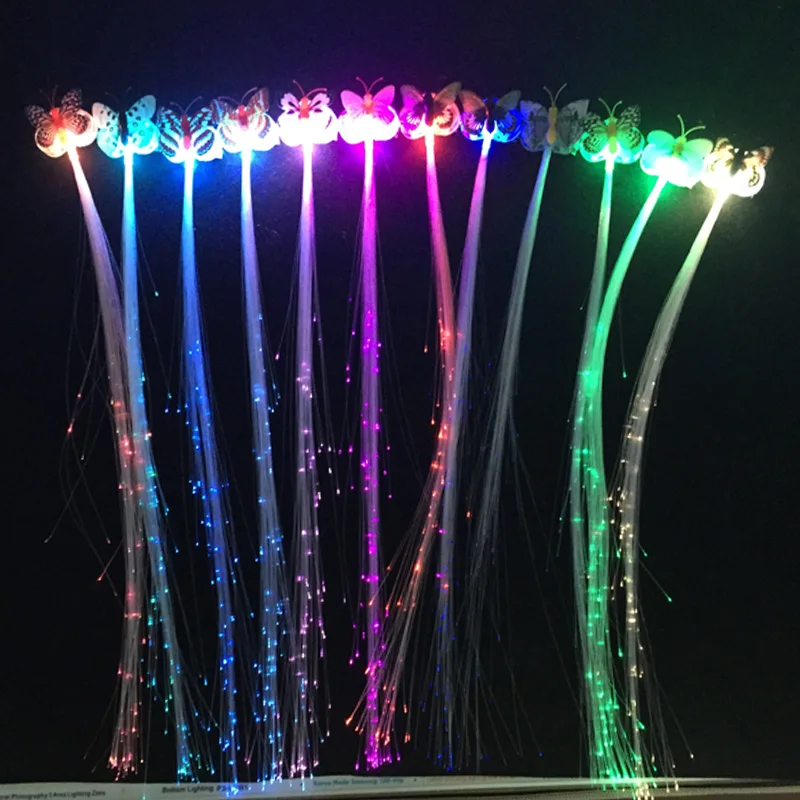The image features a line of ten butterfly-shaped objects, each illuminated by vibrant, individual spindles of light that extend downward in a tail-like fashion, resembling delicate, colorful streamers. The butterflies span a spectrum of hues, including fiery reds, blues, violets, magentas, pinks, greens, and yellows. Each butterfly appears to emit around 15 light strings, dotted with neon-colored points that spread out from the center, creating a mesmerizing visual effect against a completely black background. The floor beneath is softly illuminated by the array of colors, contrasting with a pretty white paper-like structure that lies along the bottom edge, adding an extra layer of complexity. The overall scene evokes the whimsical charm of a carnival prize, with an intricate and playful design that captivates the viewer despite the pixelation and noise in the dark, slightly blurry photo.